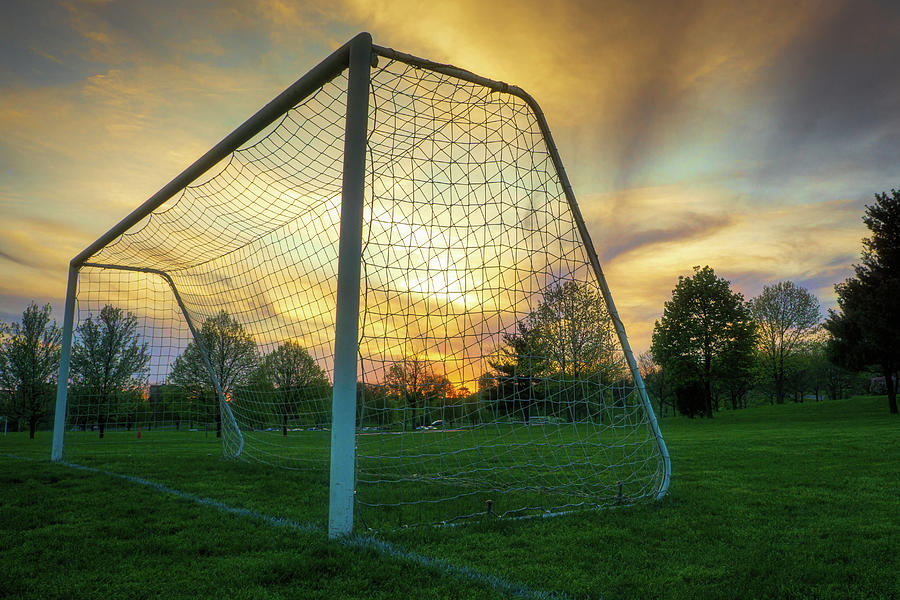The photo captures a solitary soccer net at sunset, viewed from a low angle, showcasing the front right post and netting as they stretch to the left and background. The scene is bathed in a striking blend of orangey, golden-yellow, and fire-red hues from the setting sun, which beams from behind darker gray clouds, casting a beautiful glow across the sky. The lush, dark green grass contrasts vividly with the colorful sky, highlighting the well-kept park where the goal stands. In the background, a scattering of trees frames the image, alongside a parking lot with a few parked cars. A white chalk line marks the ground in front of the goalpost, adding a touch of detail to this professionally composed shot.